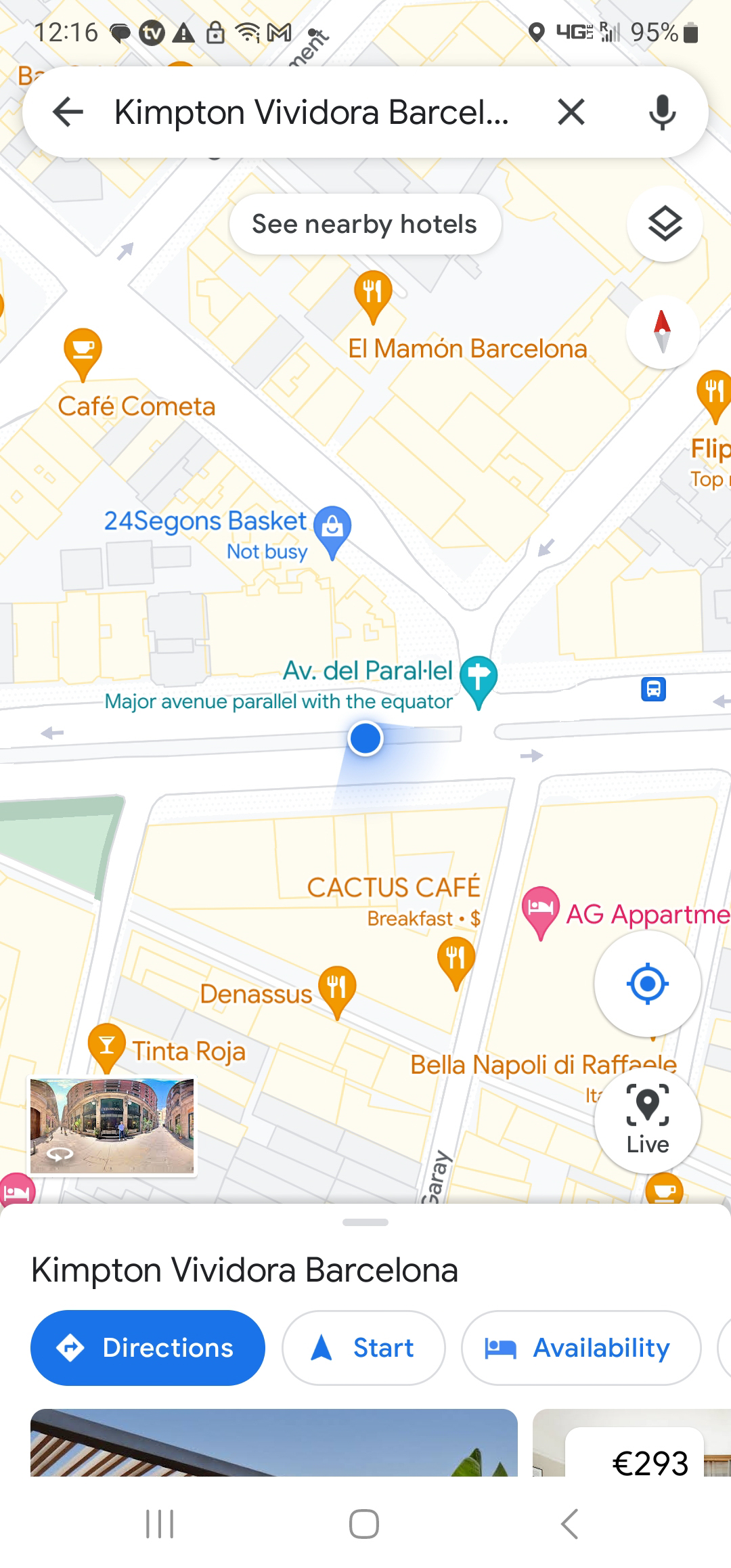A smartphone screen displays a map interface similar to Google Maps or Apple Maps. At the top, the search bar reads "Kimpton Viva Dora Barcelona..." The map is populated with various location markers such as "Cactus Cafe Breakfast" denoted by a single dollar sign, "Tinta Roja," and "AG Apartment." A "See Nearby Hotels" banner stretches horizontally across the top.

The map itself features white streets with light yellow building outlines. In the bottom left corner, a tiny street view image of one of the marked locations is visible. At the bottom center of the screen, the text "Kimpton Viva Dora Barcelona" is accompanied by three prominent buttons: "Directions," "Start," and one featuring a bed icon indicating availability.

Additionally, there are two partially visible images at the bottom. The bottom right corner displays a symbol for euros followed by "293."